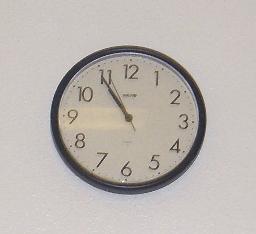A circular wall clock is prominently displayed, featuring a sleek black rim complemented by a silver bezel that adds a touch of elegance. The clock's face is covered by a clean, clear plastic crystal, ensuring visibility of the time. The clock has a pristine white background, clearly marked with black numbers from 1 to 12, and hash marks indicating the individual minutes between the numbers. Minute and hour hands point precisely to 10:54, and the second hand is just shy of the 57th second. Above and below the center point of the clock face, there are small inscriptions that are too diminutive to be legible. This timepiece is mounted on what appears to be a gray wall, though the color may actually be white.